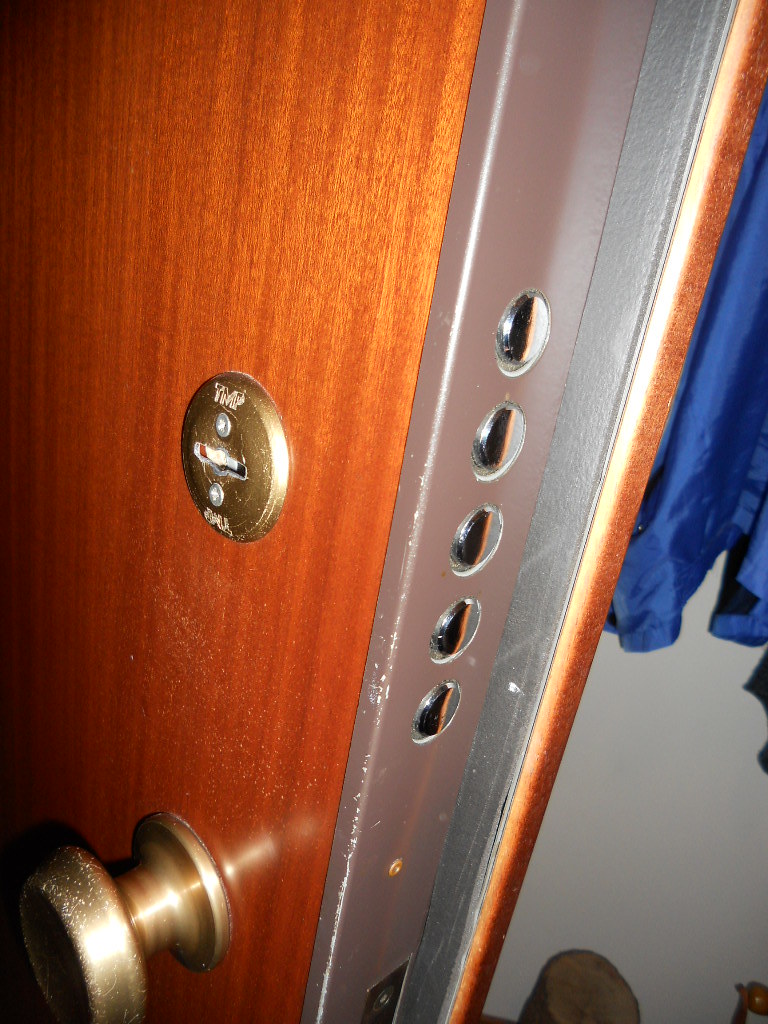The photograph showcases an up-close view of a door, highlighting its intricate details and surroundings. The door, made of cherry wood with vertical grain patterns, features a bronze-colored doorknob located in the bottom left corner. Just above the doorknob is a similarly hued brass key plate with a central slot for a key. Both the doorknob and key plate display signs of wear, with scuffed and chipped areas revealing a silver beneath the bronze.

The door's edge is framed with a thin strip of silver metal, which shows signs of wear and scrapes. Embedded within this metal frame are multiple small holes, including five circular mechanisms designed to secure the door with platinum silver locking components. Toward the bottom of these mechanisms, a hole accommodates the doorknob’s latch.

In the background, to the right of the door, there are hints of a closet or storage area. This space features hanging items, including a dark blue windbreaker and potentially other blue garments. Scattered shoes are visible on the floor beneath the hanging coats.